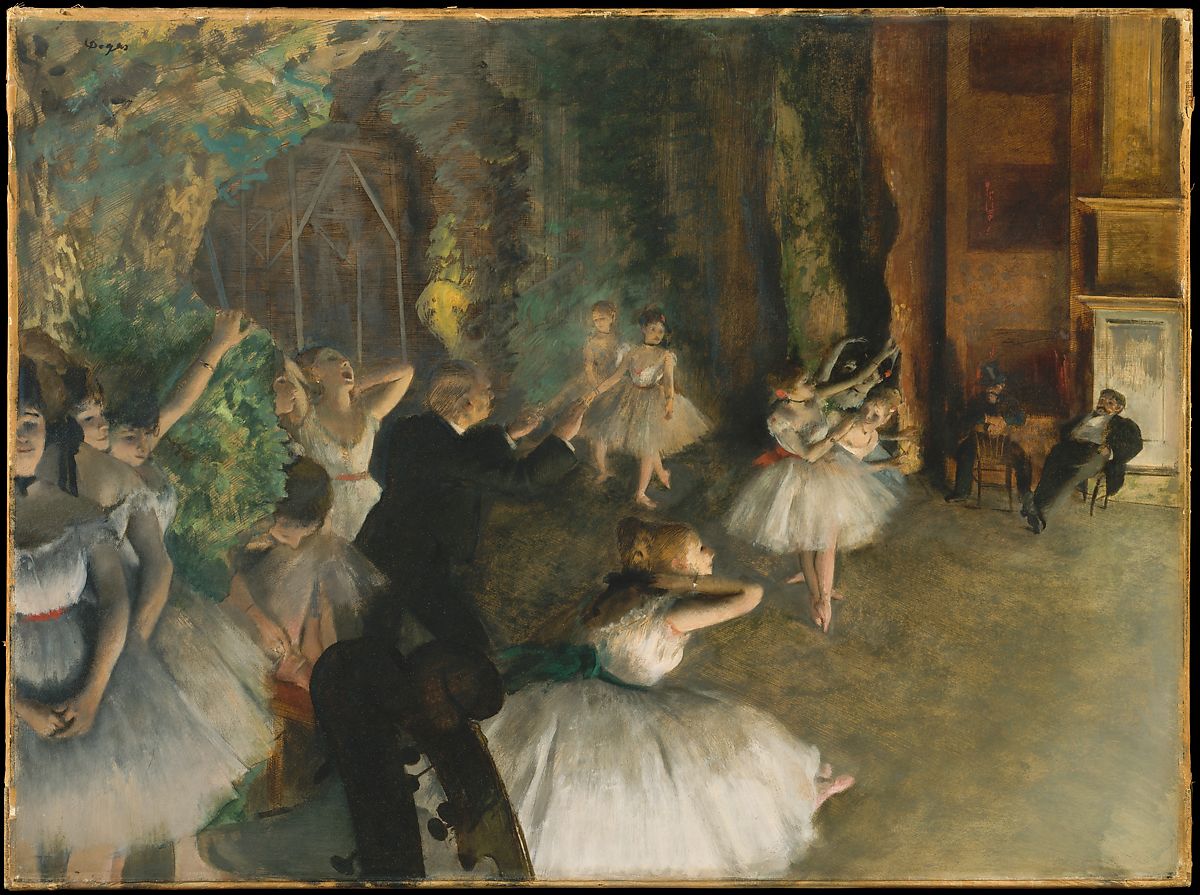This detailed photograph of an oil painting captures a dynamic ballet scene set on a stage with wooden walls, evoking a lively theater atmosphere. The backdrop on the back left features greenery, suggesting a scene setup. Prominently positioned in the center of the image are numerous ballet dancers in various expressive poses: some on the right with arms gracefully raised, others in the background with legs crossed, and one front and center appearing to be kneeling. Several dancers on the left have their arms crossed in front, with one having her left hand on the backdrop. Among them, a striking figure, who seems to be screaming with elbows crooked and hands behind her head, draws attention. In the mix, a man, possibly a conductor, stands with his arms elevated, adding to the impression of a performance in progress. Two men sit on the right, one leaning back with legs crossed, the other sitting backward on his chair, watching the dancers intently. The tops of two cello-like instruments peek into the far foreground, reinforcing the theme of a dance venue. The painting is bordered by a solid black frame with a golden edge, indicating an indoor setting suitable for an art show or a museum exhibit. The colors span a palette of black, yellow, brown, green, blue, white, gray, and tan, enhancing the rich details and layers of the composition.